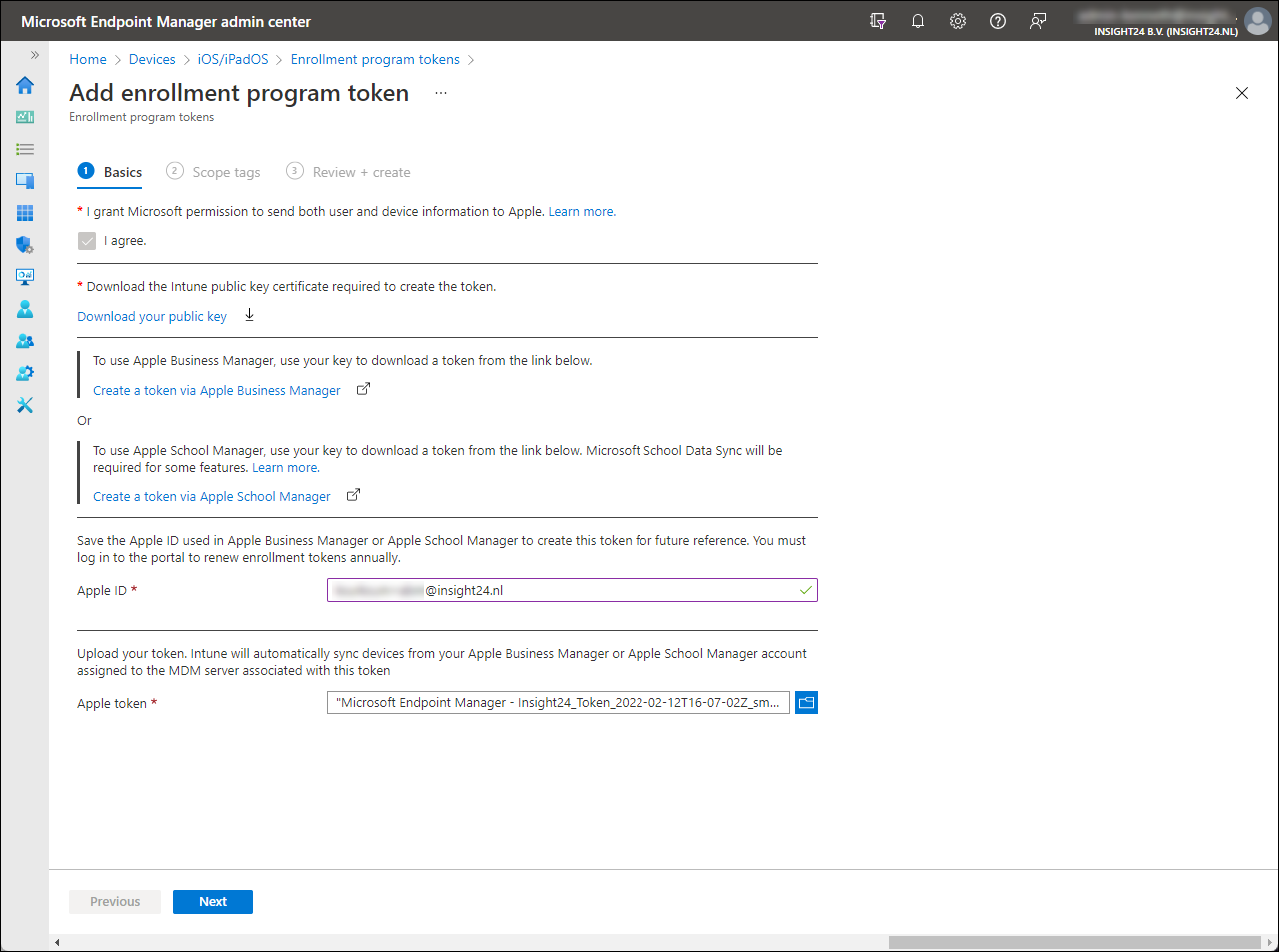**Screenshot Description: Microsoft Endpoint Manager Admin Center**

The screenshot is taken from the Microsoft Endpoint Manager Admin Center, as indicated by the black banner at the top with white text. Below this banner, the page has a clean, white background.

At the top of the content area, there's a breadcrumb navigation trail displayed in small blue letters, guiding users through the interface:
- Home > Devices > iOS/iPadOS > Enrollment Program Tokens

On the left-hand side of the screen, a vertical menu bar features various icons:
1. Home
2. A list icon with three lines and bullets
3. Copy icon
4. Shield icon (likely for security-related features)
5. People icon
6. An individual person icon
7. Settings icon
8. Tool repair icon

In the central part of the screenshot, bold black text indicates the primary task: "Add Enrollment Program Token". Below this, the section title "Enrollment Program Tokens" is displayed.

A blue icon with the number "1" signifies the active step, labeled "Basics". 

Here are the detailed descriptions and instructions displayed on the page:
- A statement granting Microsoft permission to share both user and device information with Apple, accompanied by a checkbox and the text: "I agree."
- Instructions to download the Intune Public Key Certificate, which is necessary to create the enrollment token.
- Guidance on using Apple Business Manager with a key to download the token from an embedded link.
- A final reminder to save the Apple ID and use either Apple Business Manager or Apple School Manager to create the token for future reference, with a note about the necessity of logging into the portal for token renewal. 

At the bottom, there is a field for entering the Apple ID.

This detailed description provides a comprehensive overview of the components and instructions seen in the Microsoft Endpoint Manager Admin Center screenshot.